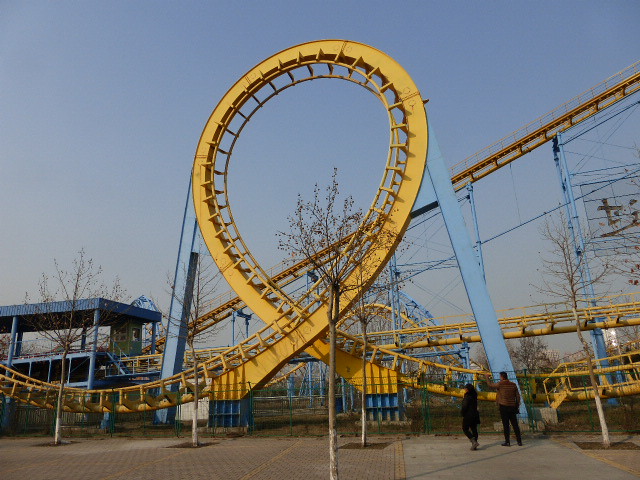In this detailed photograph of an amusement park, the central focus is a large and striking roller coaster, primarily colored in dark and yellow with light blue support beams. Dominating the foreground is an impressive 150-foot-tall, inverted loop, which serves as a captivating focal point. A long ascending track runs from a building in the bottom left corner towards the top right, further emphasizing the ride's grandeur and height. Behind the ascent, another inverted helix loop is visible, reinforcing the roller coaster's complex design.

In the bottom right corner, two individuals—a male and a female—stand near one of the blue support structures, seemingly admiring the structure. The male is pointing up at the roller coaster, which suggests a sense of awe and enthusiasm. The scene is set against a clear sky, possibly in the morning, as there is no visible sun and the park appears empty with no other visitors around. Sparse trees can be seen in the background, enhancing the open, unoccupied feel of the park. The overall impression is one of a thrilling, towering roller coaster in a calm and quiet amusement park setting.